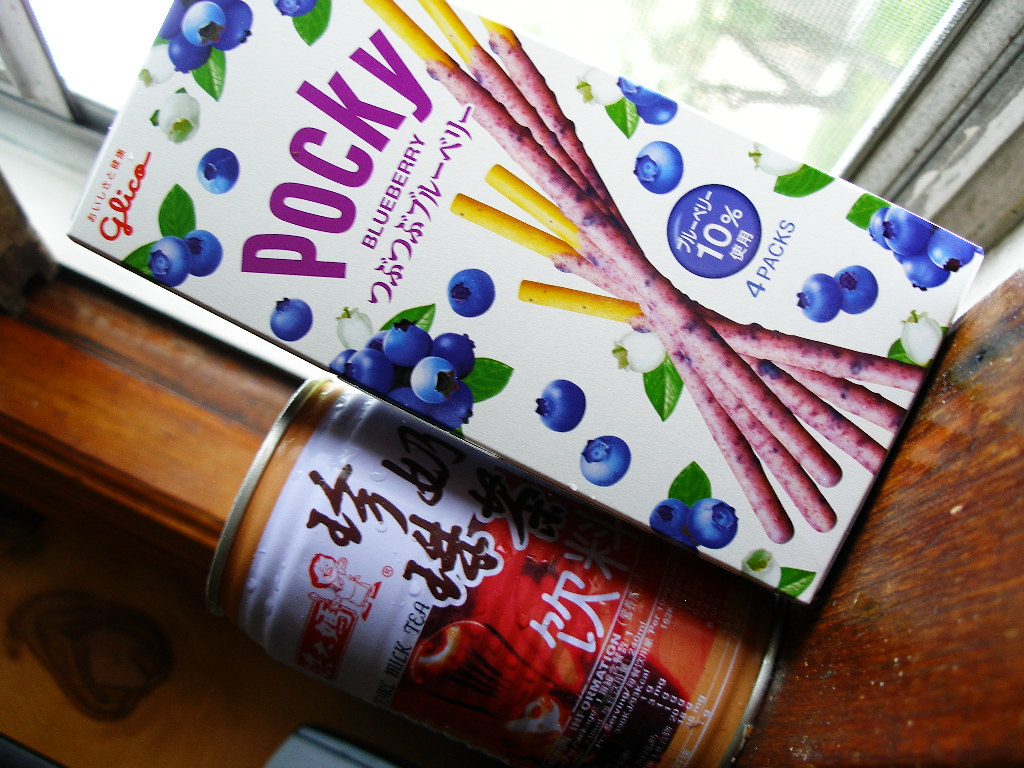In this somewhat tilted image, we see a wooden windowsill beneath a window. Prominently featured are two items on the sill: a box of Pocky Blueberry and a can of something with partially visible Asian writing. The Pocky box is vividly detailed with images of blueberries and dipped sticks, alongside text that says "Glyco" at the top and "POCKY" in purple letters in the middle, followed by "Blueberry." Additionally, there's a blue circle on the box indicating "10%" and further Asian writing below mentioning "four packs." The precise nature of what's in the can remains unclear, but it appears to be a tea or similar beverage, with only the letter "T" discernible among the Asian characters. The entire scene, slightly rotated, suggests an informal, somewhat casual still life composition centered on these snack items.